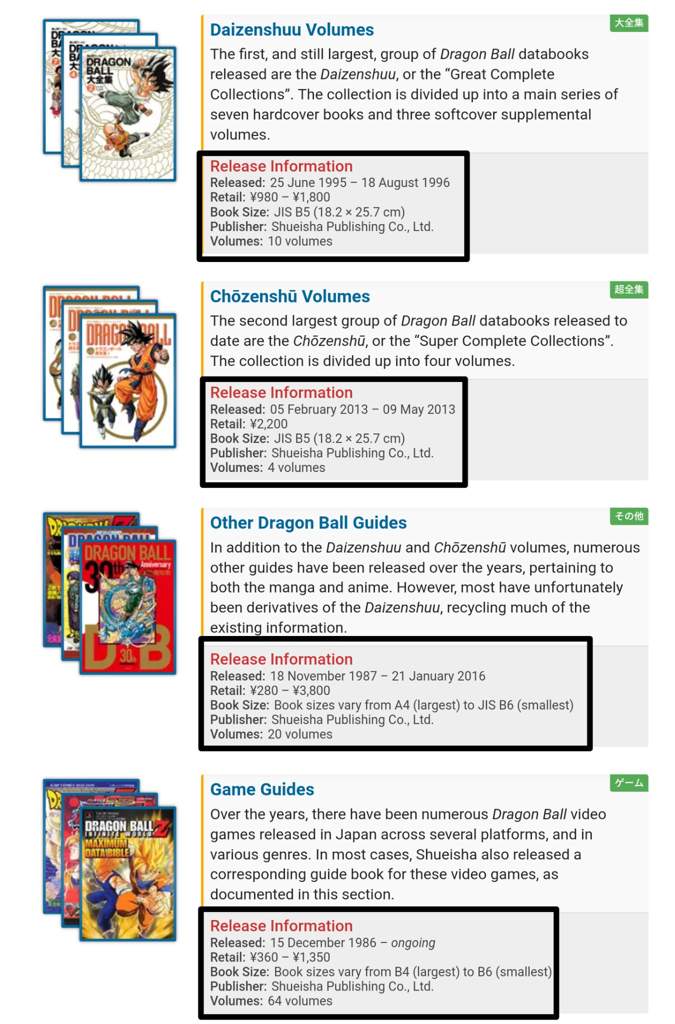The image depicts a detailed section of a manga-focused website, specifically related to Dragon Ball publications. It showcases various volumes categorized into four distinct entries: **Daisenshu** volumes, **Chozenshu** volumes, other Dragon Ball guides, and game guides. On the right side of each entry, there are images of stacked magazine or book covers, with three stacked for each category, providing a visual representation of the publications.

At the top of the image, the first entry is dedicated to the **Daisenshu** volumes, described as the primary and largest collection of Dragon Ball data books. Referred to as the "Great Complete Collections," this series comprises seven hardcover books and three softcover supplemental volumes, totaling ten volumes. Below this, additional details about the Daisenshu volumes include:

- **Release Dates**: June 25, 1995, to August 18, 1996
- **Retail Value**: 980 to 1800 JPY
- **Book Size**: GIS B5 format, 18.2 x 25.7 cm
- **Publisher**: Shueisha Publishing Company Limited

These specifics are organized in a section labeled "Release Information," prominently highlighted by a manually added black rectangle against the website's light beige background. This highlighting format is consistently applied to all four entries, indicating that the additional information has been manually emphasized for clarity. The comprehensive details and the structured layout of the image provide a thorough overview of the Dragon Ball guide collections available.